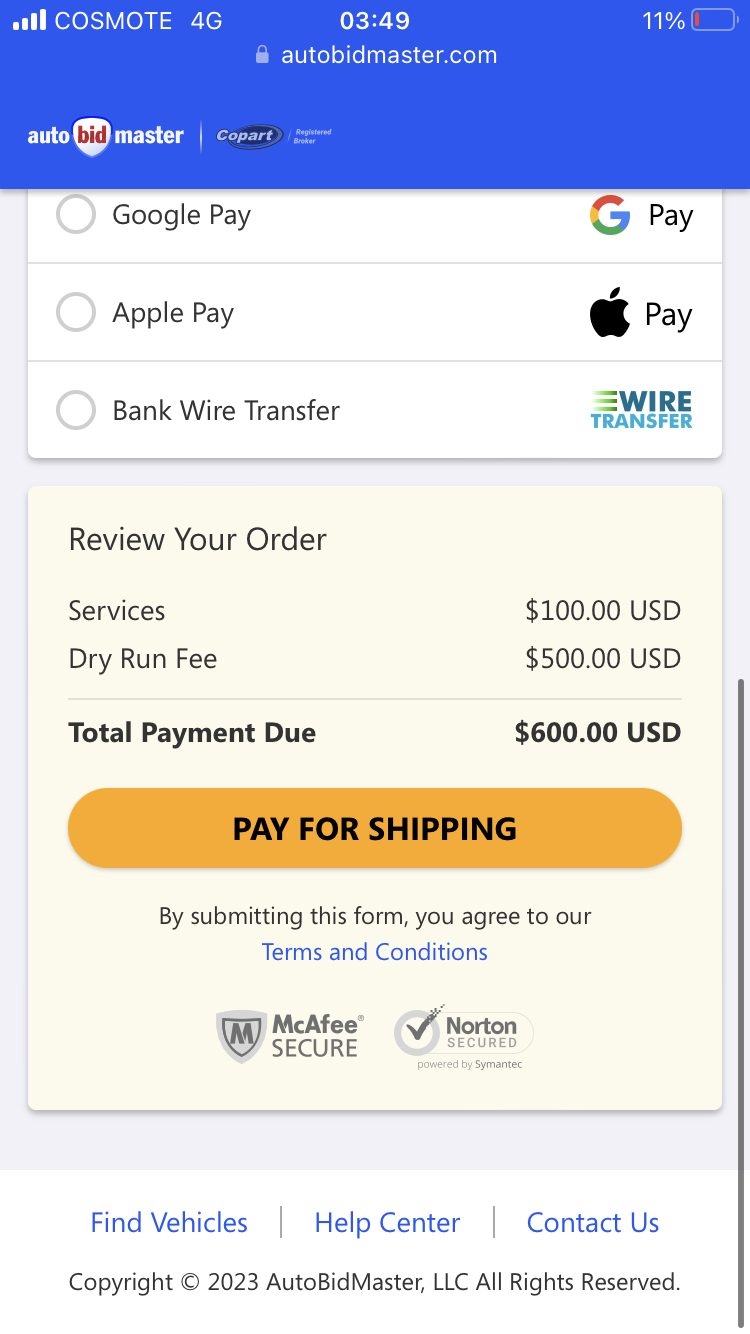This screenshot captures a mobile phone display showcasing a webpage from the website AudioBidMaster.com. At the top, near the center, there's a lock icon indicating a secure connection. Above the website URL, the time is displayed as 3:49 PM on the right, next to a nearly depleted battery at 11% in the red zone. The top left features a signal bar and the network name "Cosmo 4G".

The webpage layout includes a blue header, while the body of the page is light gray. Two charts dominate the content. The first chart lists various payment options such as Google Pay, Apple Pay, and bank wire transfer. The second chart details the total order, which includes a $600 payment composed of $100 for services and $500 for a drive run fee.

Security features are highlighted with the presence of McAfee Secure and Norton Secure logos at the bottom of this section. Below these logos, an orange 'Pay for Shipping' button is prominently displayed. Nested between the 'Pay for Shipping' button and the security icons is a 'Terms and Conditions' section.